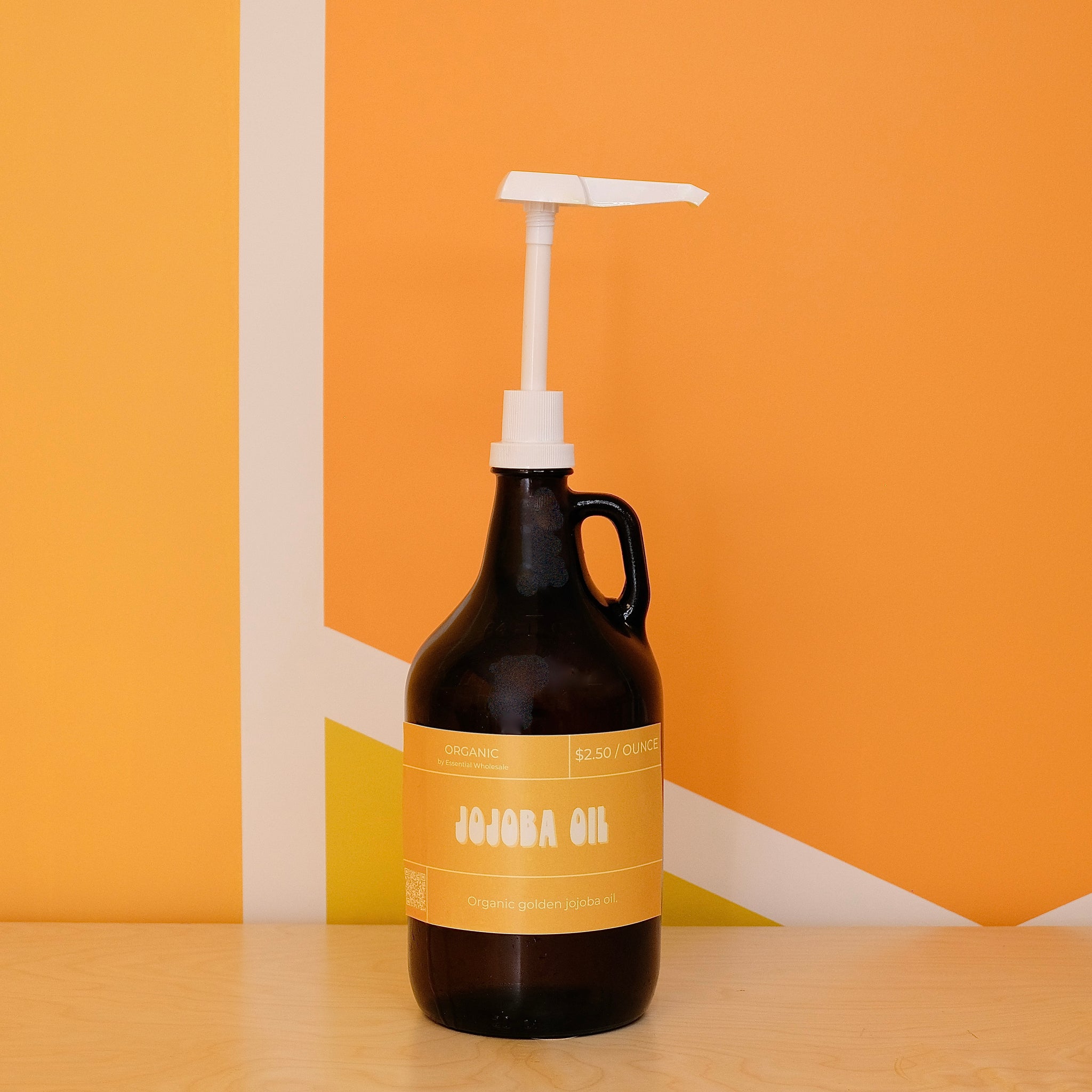The image depicts a room with a table, featuring a prominently placed product—a large, black plastic jug of organic Jojoba oil. The jug, which holds 32.5 ounces, has an extended white pump on the top and a bold orange label with the text "Jojoba Oil" in white lettering. The label is detailed, although some smaller text on it is unreadable. The jug rests on a brown counter, which complements the distinctive geometric wallpaper behind it. This wallpaper features several shades of orange segmented by a white stripe that extends at an angle, creating a striking backdrop that makes the jug stand out. The repeated orange hues and geometric patterns, along with the unique product presentation, give the room an intense, albeit somewhat overwhelming, visual aesthetic.